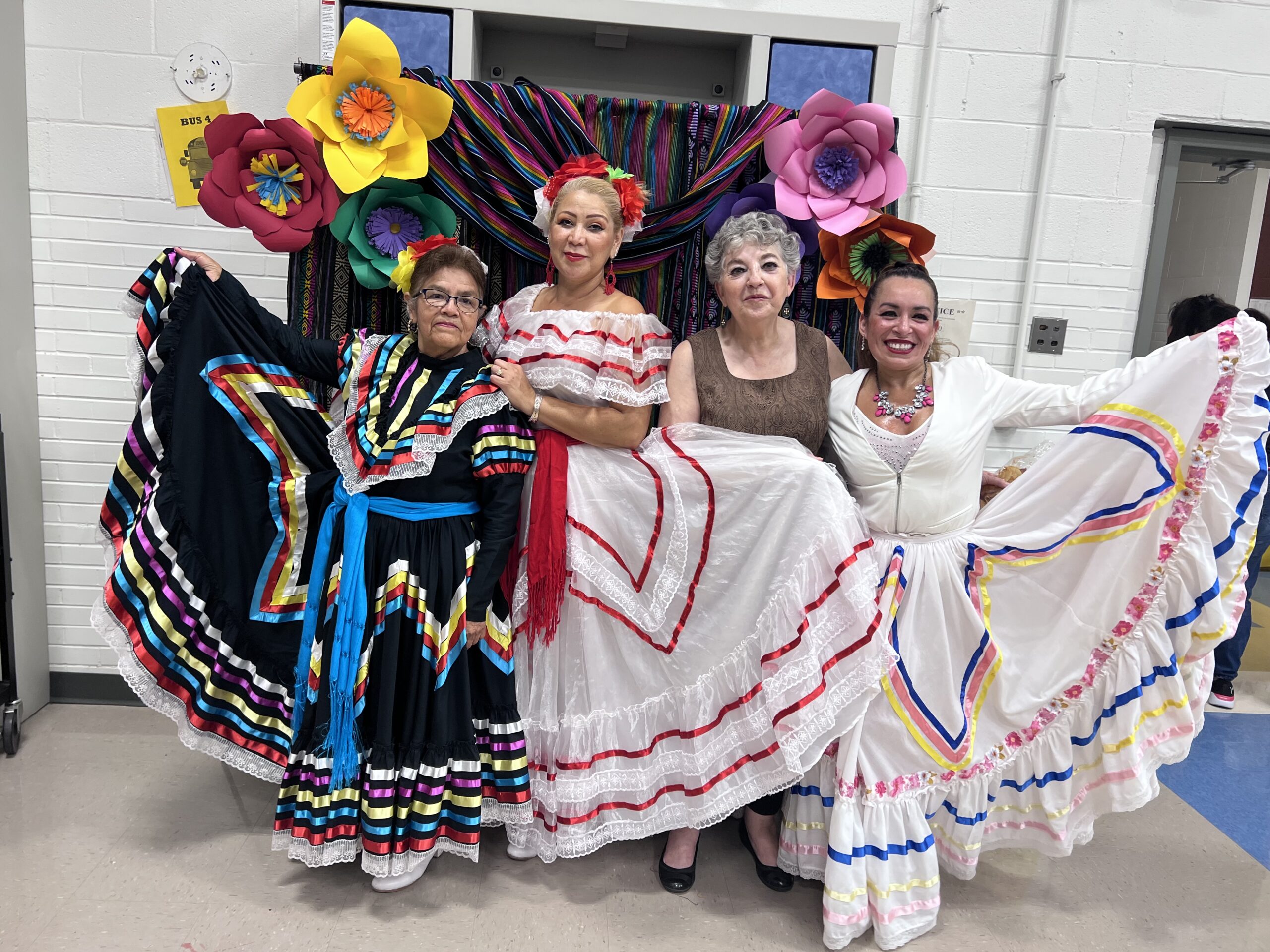In the image, four individuals are dressed in vibrant Hispanic cultural attire, indicative of a festive celebration. The woman in the center wears a striking long white dress accented with red trim, and her hair is adorned with flowers in the colors of red, green, and white. To her right, another woman is dressed in a predominantly white gown embellished with blue, pink, and yellow petal-like designs at the bottom. On the far left, a woman is holding up her primarily black dress, which features elaborate petal patterns in white, purple, yellow, light blue, and red lines. The backdrop behind them is festooned with flowers in pink, yellow, red, and green hues, seamlessly complementing the colorful attire and enhancing the overall festive atmosphere.